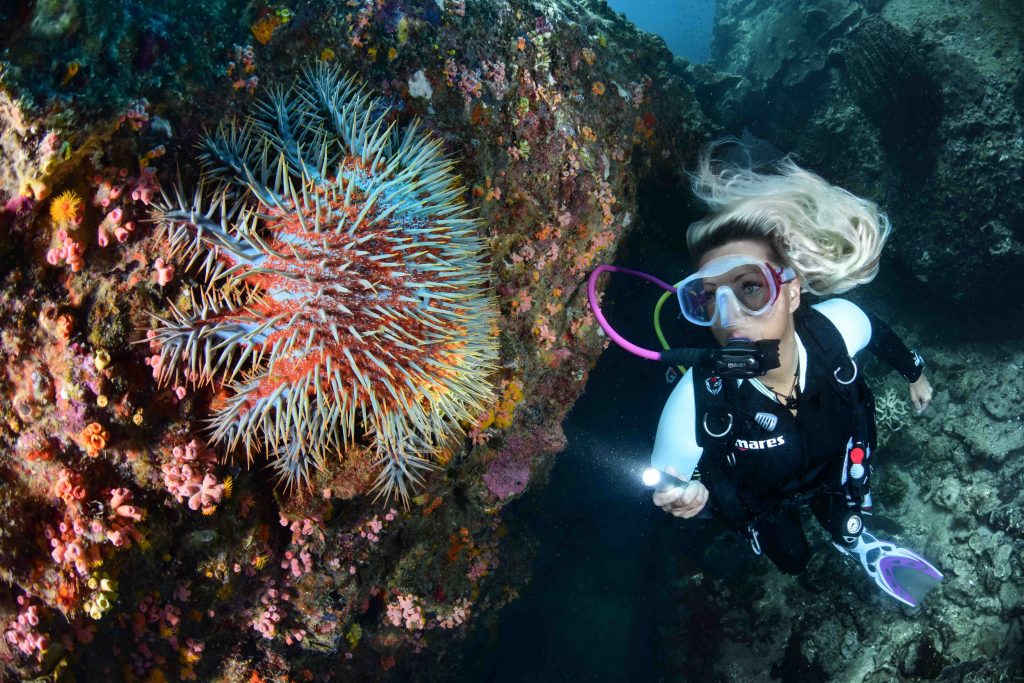The underwater photograph showcases a clear blue scene teeming with vibrant marine life and rocky formations. On the right side of the image, a female scuba diver, wearing black and white scuba gear, a mask, and a breathing regulator connected to her oxygen tank, is captured mid-dive. She has long blonde hair with visible brown roots, and is holding a flashlight that illuminates the left side of the image. Her fins are colored teal and purple. The diver's gaze and flashlight focus on a striking red and blue spiky organism, featuring an oval-shaped body with multiple arm-like extensions covered in blue spikes. Surrounding this creature, a variety of brightly colored corals and sea anemones in shades of pink, green, and orange decorate the gray and brown rocky landscape, creating a stunning underwater tableau.